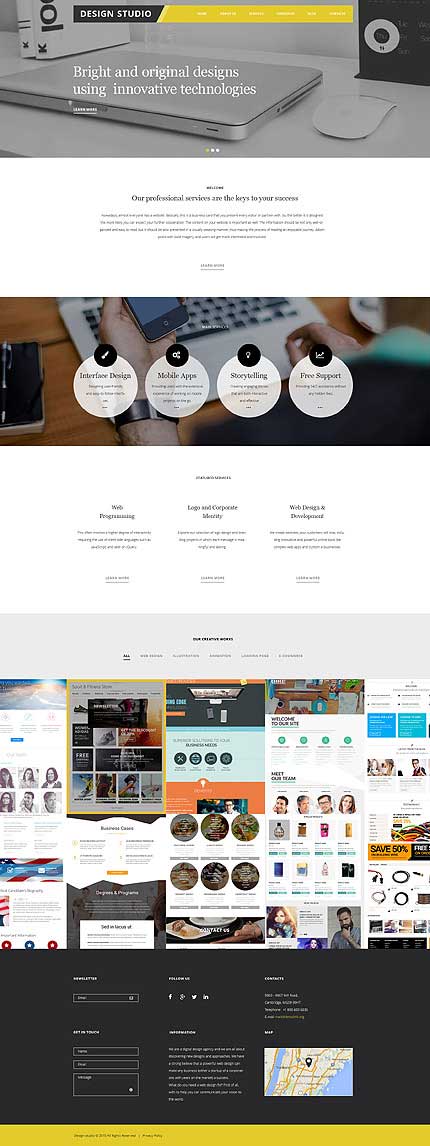The image at the top features a small gray box displaying a desktop setup with a tablet, mouse, and speaker. There is some white text within this box that is unreadable. Below this, a white space with blue text is visible. Following this, another image shows a phone, a computer keyboard, and four circles with black icons above them. These icons depict a pencil, a square, a plus sign, and a line. 

Further down, there is more blue text on a white background, followed by a light blue box containing additional text. Underneath this, several drop-down menus are visible, showcasing a variety of products, people, and places. 

At the bottom of the overall image, there is a wide, dark gray box that includes a small map in the lower-left corner, with another section below that colored yellow.